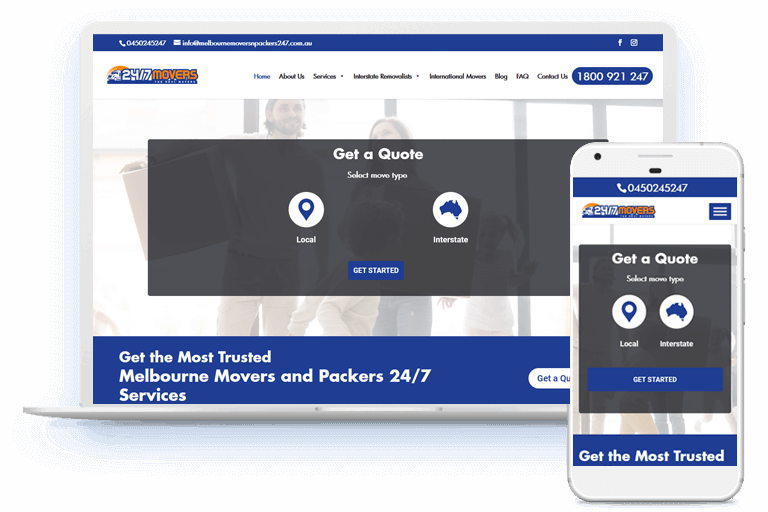This image showcases a mock-up of a website for "24-7 Movers," presented on a laptop and a smartphone. The laptop is positioned in the background on the left side, while the smartphone is slightly overlapping it in the foreground on the right. 

On both devices, the website features the "24-7 Movers" logo in the upper left corner, which is designed in shades of orange, blue, and white. The navigation menu includes options for Home, Ballot Services, Interstate Removals, International Moves, Blogs, FAQ, and Contact Us. Adjacent to the menu is a prominently displayed phone number, 1-800-921-247, on a blue header. 

In the background of the main content area, there is a faint image of a man and a woman. Overlaid on this image is a large rectangle containing interactive elements such as a "Get a Quote" button and two map pins – one labeled "Local" in a white circle, and another labeled "Interstate" with an icon of Australia. There is a blue "Get Started" button also present in this section.

At the bottom of the screen, a footer text reads, "Get the most trusted Millburn movers and packers 24-7 services," followed by a "Get a Quote" call-to-action. The smartphone display mirrors these elements but in a format tailored for mobile viewing, showcasing the adaptive and responsive design of the website.

The overall design dynamically adjusts to the device used, ensuring an intuitive and consistent user experience across different platforms.